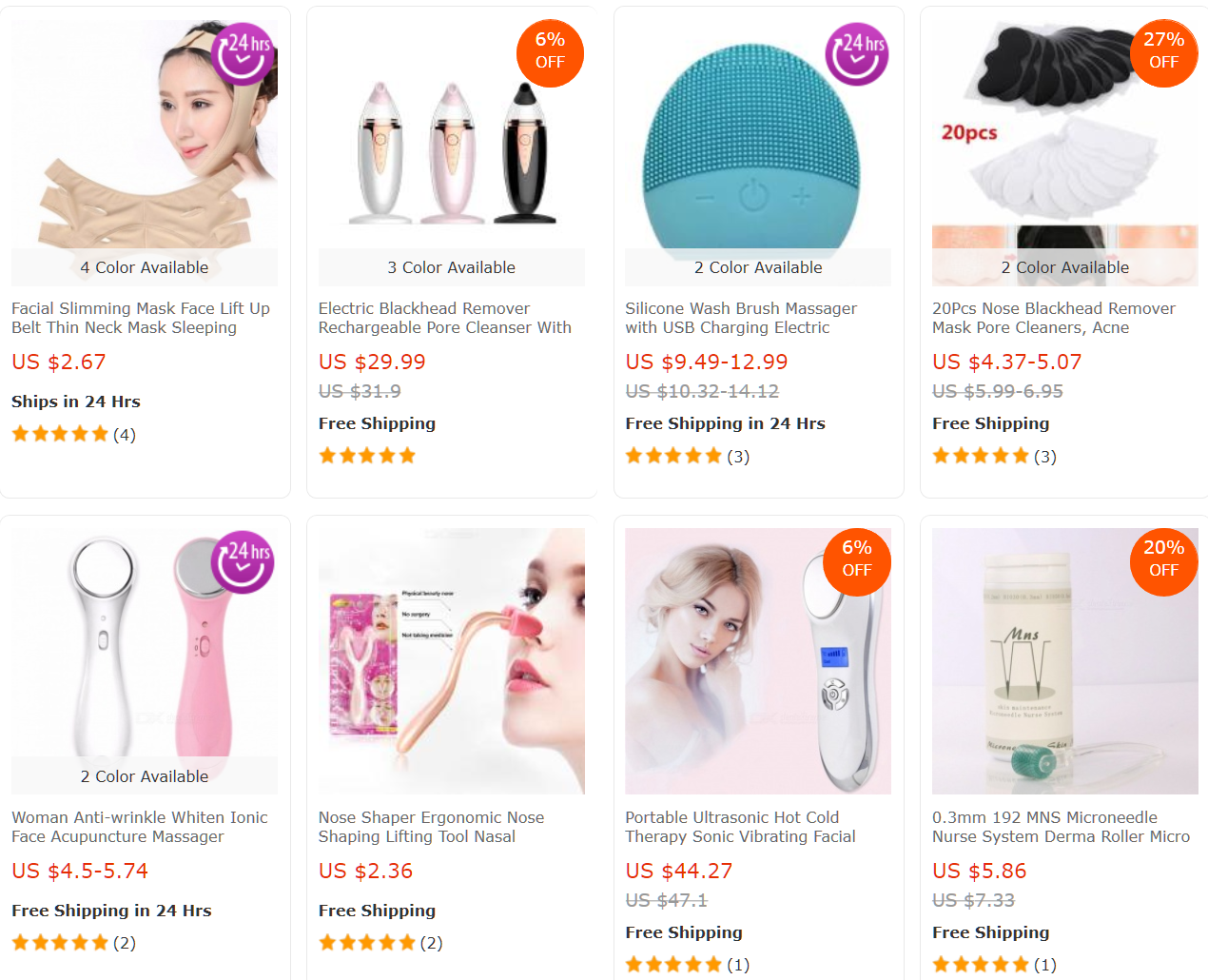In this image, we are looking at a screenshot of a shopping website set against a solid white background. The layout features eight items for sale, arranged in two rows of four. 

Starting from the lower left, the first item is a women's anti-wrinkle ionic face acupuncture massager, available in two colors: white and pink. The pink massager is highlighted with a purple circle icon that reads "24 hours" in white text, indicating fast shipping. The price for this item is listed in red as US $4.50 to $5.74, with a note in small dark black text beneath it stating "Free shipping in 24 hours." It has received a five-star rating from two reviews.

To the right of this item is a nose shaper, an ergonomic nose shaping and lifting tool. The product image features an illustration of a female with the apparatus attached to her nose.